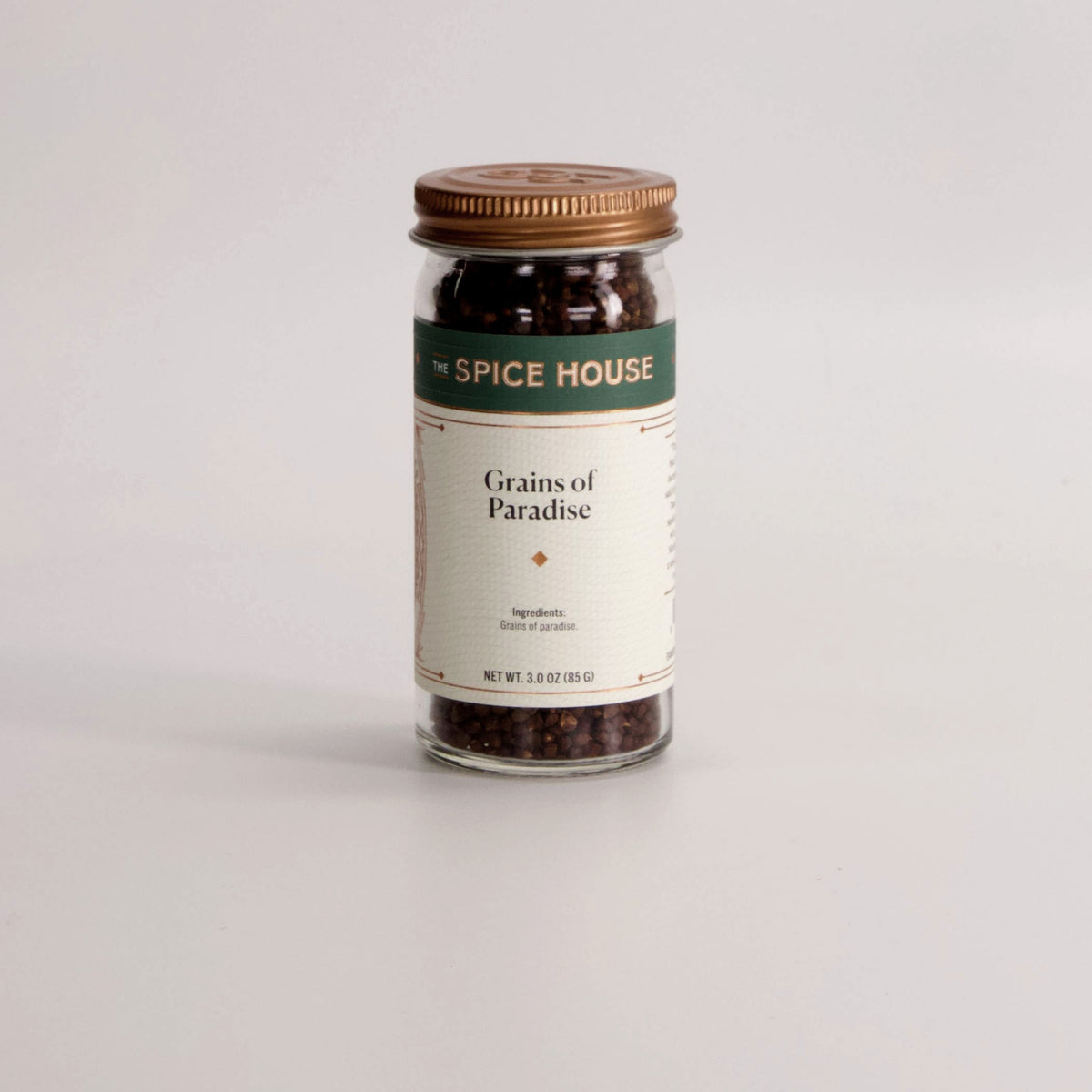This is a detailed photograph of a small, clear glass bottle containing a spice called Grains of Paradise. The bottle is capped with a bronze, screw-on metallic lid. The label on the front is primarily white with a green stripe at the top, featuring gold-colored text that reads "The Spice House." Below this, in black letters, it states, "Grains of Paradise," with a gold diamond-shaped symbol situated directly below the text. The label also provides the net weight, which is listed as 3.0 ounces (approximately 35 grams). The spices inside the bottle are dark brown and fill the bottle to the top, although their precise appearance is hard to distinguish due to the small, fine nature of the spices. Overall, the packaging is eye-catching with its contrasting white, green, and gold design elements, and the bottle casts a faint shadow on the white countertop due to the room's lighting.